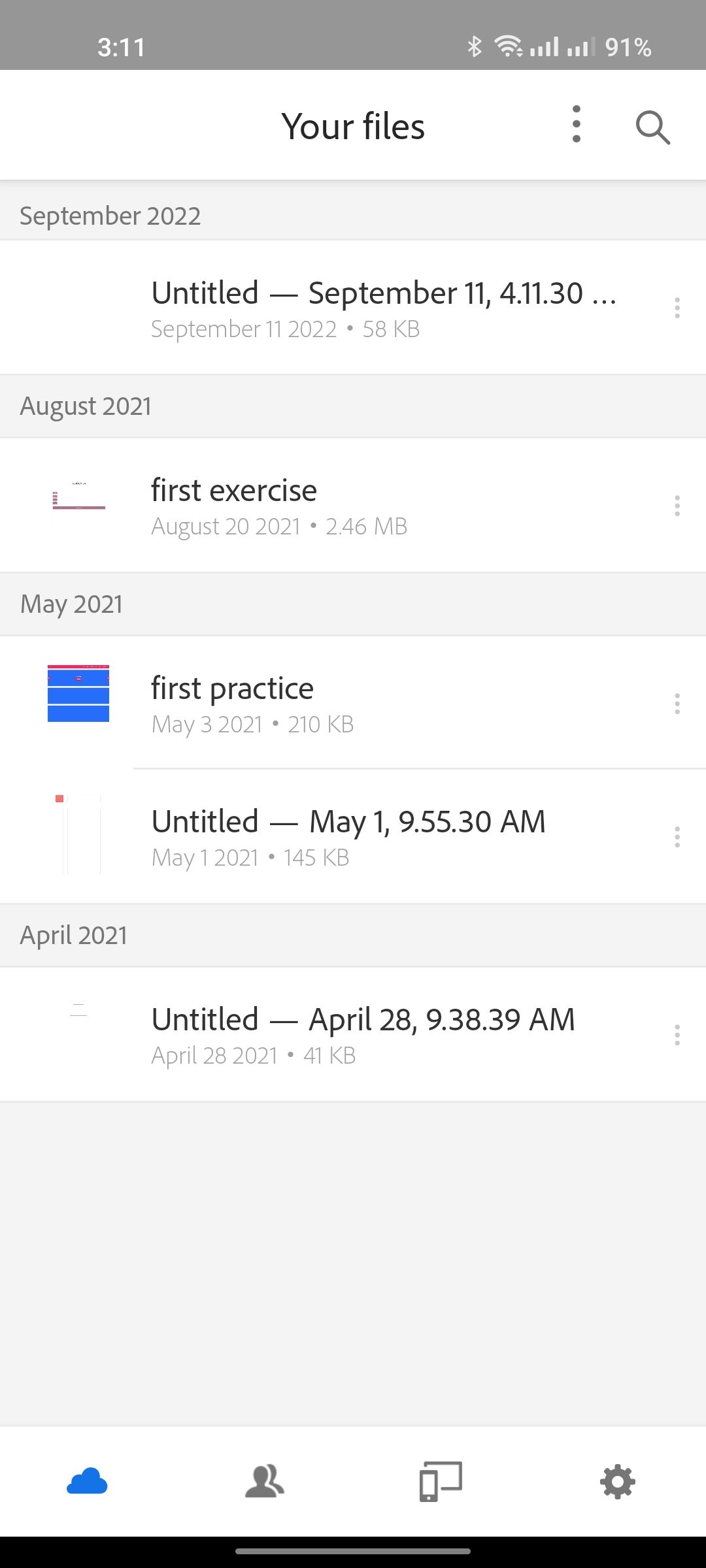The image displays a screenshot from a smartphone. The battery life indicator shows 91%, with full signal bars indicating a strong connection. The time displayed is 3:11 PM. Beneath this, a gray bar holds this information, and below it, in black text, it says "Your Files.” 

A vertical list of file entries follows, each detailed with attributes such as name, date, and size:

1. A light gray box labeled "September 2022" is prominent.
2. An entry titled "Untitled" dated September 11th with a timestamp of 4:11:30, followed by an ellipsis, shows a size of 58 KB. The complete file detail reads "September 11th, 2022, 58 KB".
3. Another section labeled "August 21" in gray color contains the entry "First Exercise" dated August 20th, 2021, with a size of 246 MB.
4. The "May 2021" section in gray includes an entry named "First Practice," featuring a blue icon with red horizontal stripes, dated May 3rd, 2021, at 210 KB.
5. An entry titled "Untitled" listed under May 1st, with the specifics "9:55:30 AM, May 1st, 2021, 145 KB", features an icon resembling a white, long, vertical box.
6. Another "Untitled" entry dated April 28th at 9:38:39 AM is also included, situated within a larger, empty gray box.

At the bottom, several icons are positioned above a final black bar.